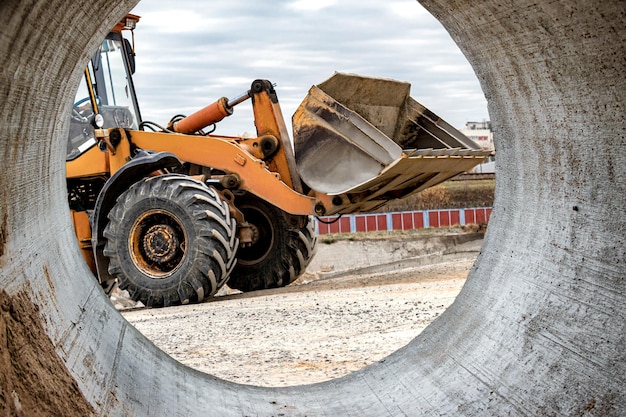This daytime image captures a scene viewed through a large cement tunnel or pipe, featuring a detailed look at construction equipment. In the foreground, circular lines can be observed on the inner surface of the tunnel, along with a pile of dirt situated in the lower right-hand corner. Looking through this cylindrical perspective, an orange bulldozer is visible, characterized by its front-end loader with an empty, upward-pointing scoop. The machine's two large tires are covered in white sand from the gravel and dirt path it rests on. The cab reveals a steering wheel but no operator is visible. Adjacent to the bulldozer, on the right, are a few brown bushes and a low-lying, partially visible wall, red and outlined in blue. Beyond the bulldozer, there appears to be a light gray building in the distance. The cloudy sky above features minimal patches of blue, adding to the overall atmosphere of the scene.